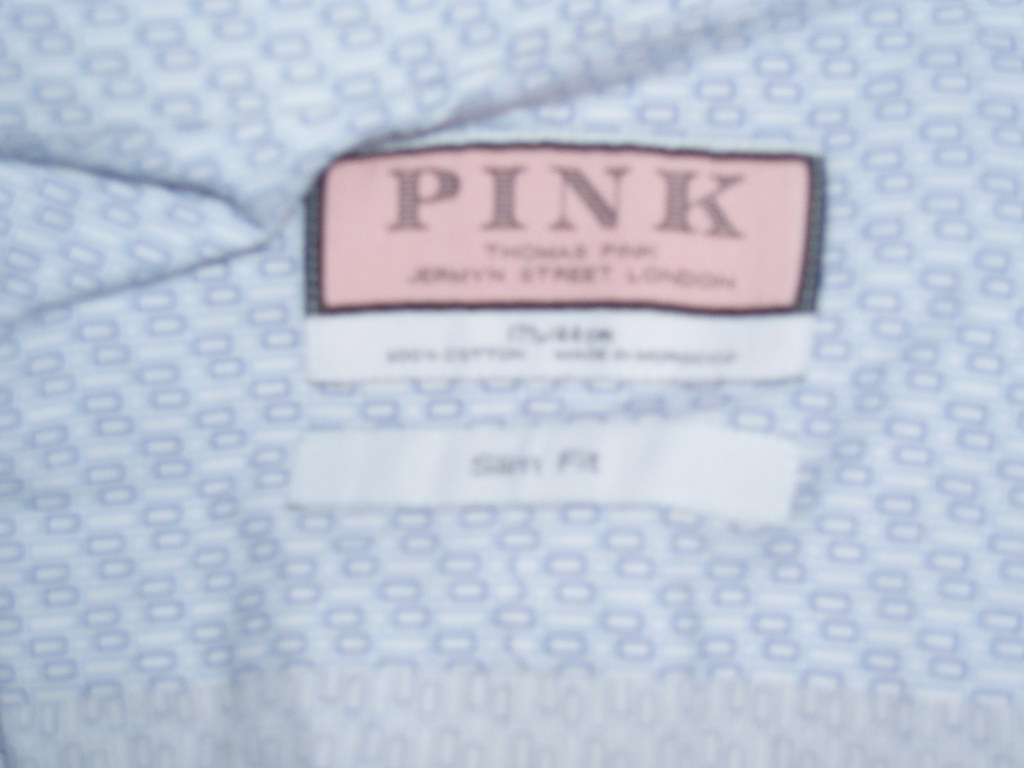The image features a light blue shirt adorned with two medium dark blue circles. The first label on the shirt is pink with black lettering and bears the brand name "Pink." Below this, there are two smaller words that are difficult to decipher, followed by three words that seem to begin with 'A' and include "Street London." Directly underneath this label is a white tag, also challenging to read, possibly containing one word followed by five words. Another white tag located slightly lower on the shirt states "Slim Fit." The overall image clarity is somewhat blurry, making some details hard to make out.